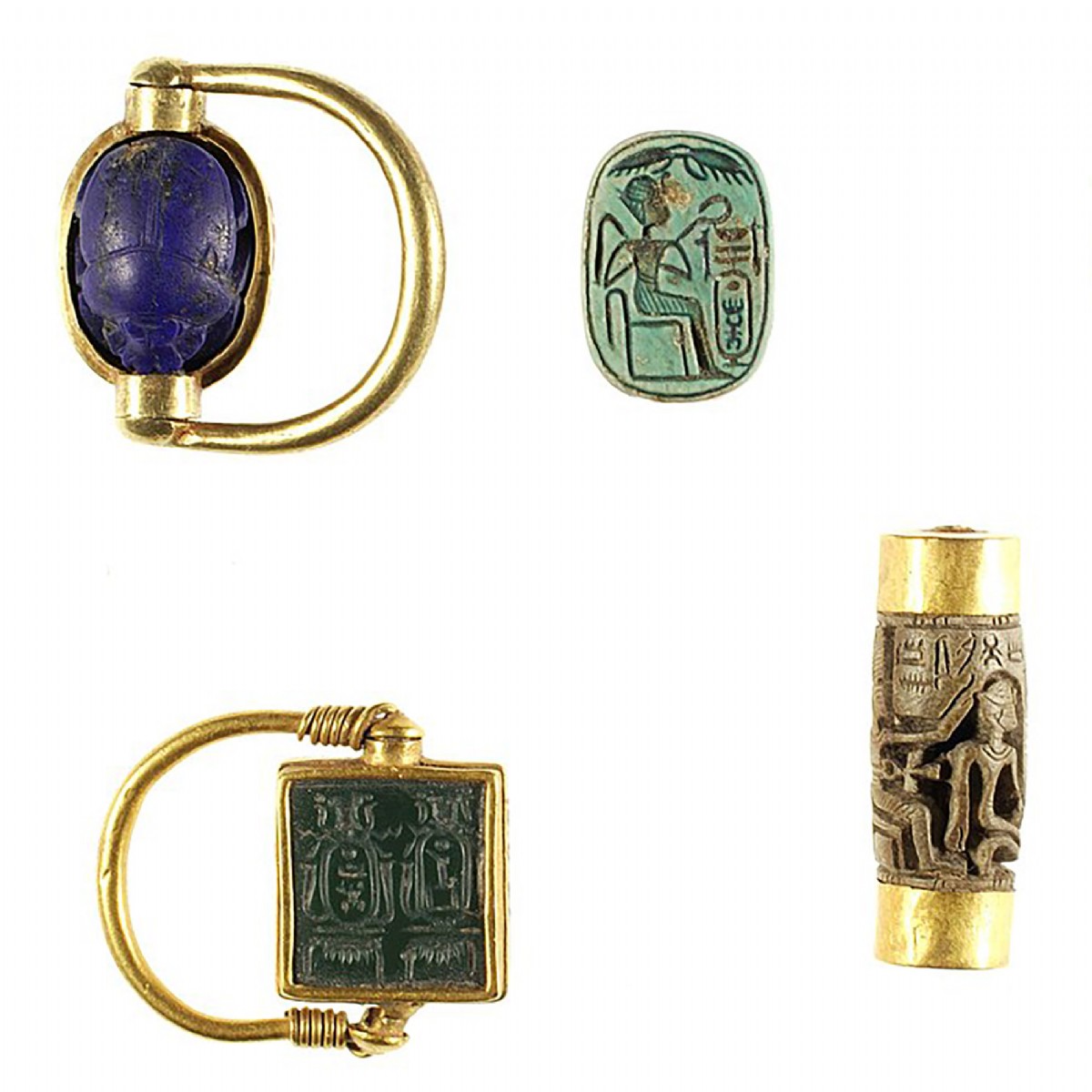The image features four distinct ancient Egerbician artifacts, each carefully detailed and steeped in rich historical significance, set against an all-white background. 

In the top left corner, there is a gold object displaying an intricate, purple-colored beetle emblem. Extending from the beetle's casing is a golden handle intricately designed, connecting at both the top and bottom. This piece appears to serve as a decorative or symbolic clasp or amulet.

To the right, a green, oval-shaped artifact showcases an engraved figure of a person seated on a chair, with what seems to be wings positioned above them, suggestive of an Egyptian influence. The item is adorned with various enigmatic symbols and intricate detailing.

On the bottom left, a golden, square-shaped piece mirrors the elaborate design of the top-left item but with wired coils connecting a golden handle to the square body. The square is detailed with engraved symbols and features, adding to its historical allure.

At the bottom right, there is a cylindrical object, brown in color with detailed engravings. This object exhibits a mix of wood and gold-toned elements, marked with more ancient symbols in shades of gray and black.

These artifacts collectively resemble ornate jewelry or ceremonial clips from a bygone era, reflecting the rich, artistic heritage of the ancient Egerbician civilization.